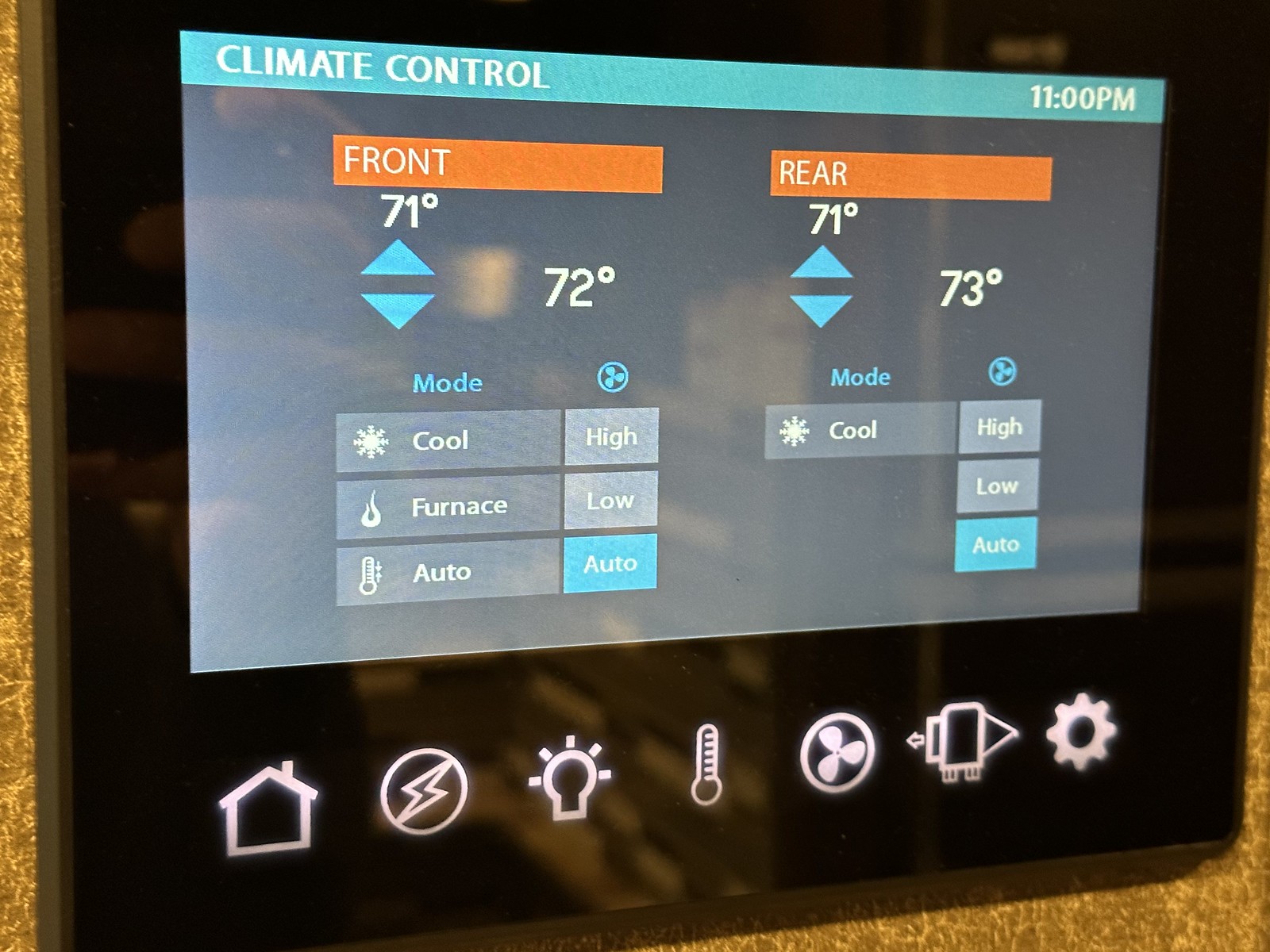This screenshot depicts a car's climate control system displayed on a touch screen interface. The design is relatively simplistic, with elements reminiscent of an iPad interface. Dominating the bottom of the screen, icons represent various car climate settings. From left to right, they include an image of a house, a circle containing a lightning bolt, a light bulb with radiating lines symbolizing sunshine, a thermometer, a fan icon, an image depicting air recycling, and a cogwheel for settings.

Across the top of the screen, there's a blue banner displaying "Climate Control" on the left side and the time, "11:00 PM," on the right side, both written in white. The rest of the screen features a black background with some minor light reflections visible.

Two prominent red banners labeled "Front" and "Rear" indicate separate climate control zones for the front and rear of the vehicle. The temperature is adjustable up and down in both zones, with current temperatures displayed. The front zone settings show "Cool" set to high, "Furnace" set to low, and "Auto" set to auto. The rear zone has a similar setup, though specifics are not fully detailed.